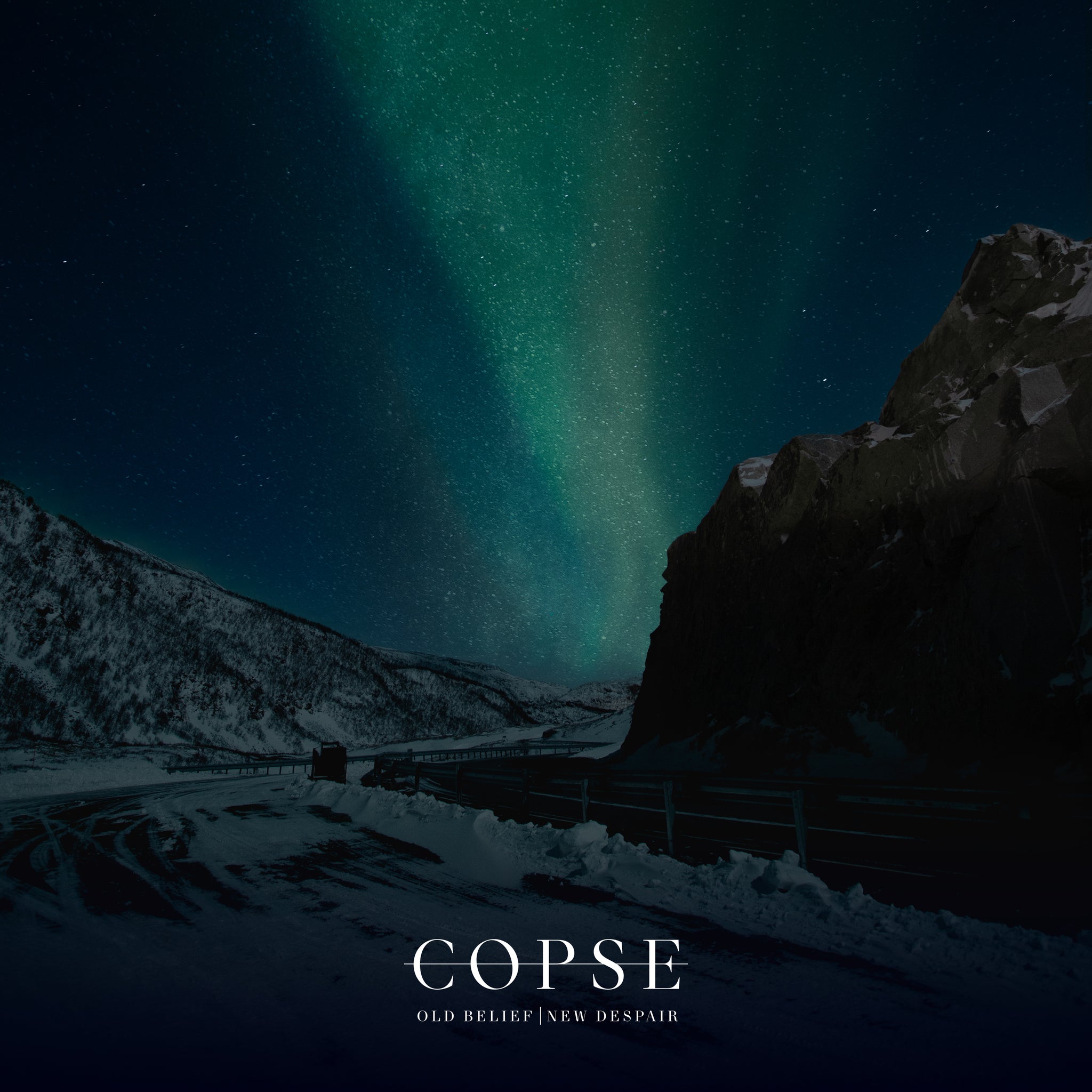In this nighttime desert scene titled "C.O.P.S.E. - Old Belief, New Despair," a majestic, rocky landscape unfolds beneath a navy-blue sky filled with twinkling stars. A striking mint-green aurora borealis trails across the sky, growing brighter and wider towards the top of the image. The barren desert terrain features sandy, gray trails that wind through a rugged area, culminating in a prominent rock formation in the upper right corner. The text "C.O.P.S.E." and "Old Belief, New Despair" are displayed prominently in a white serif font, adding an element of intrigue and hinting at deeper symbolism.